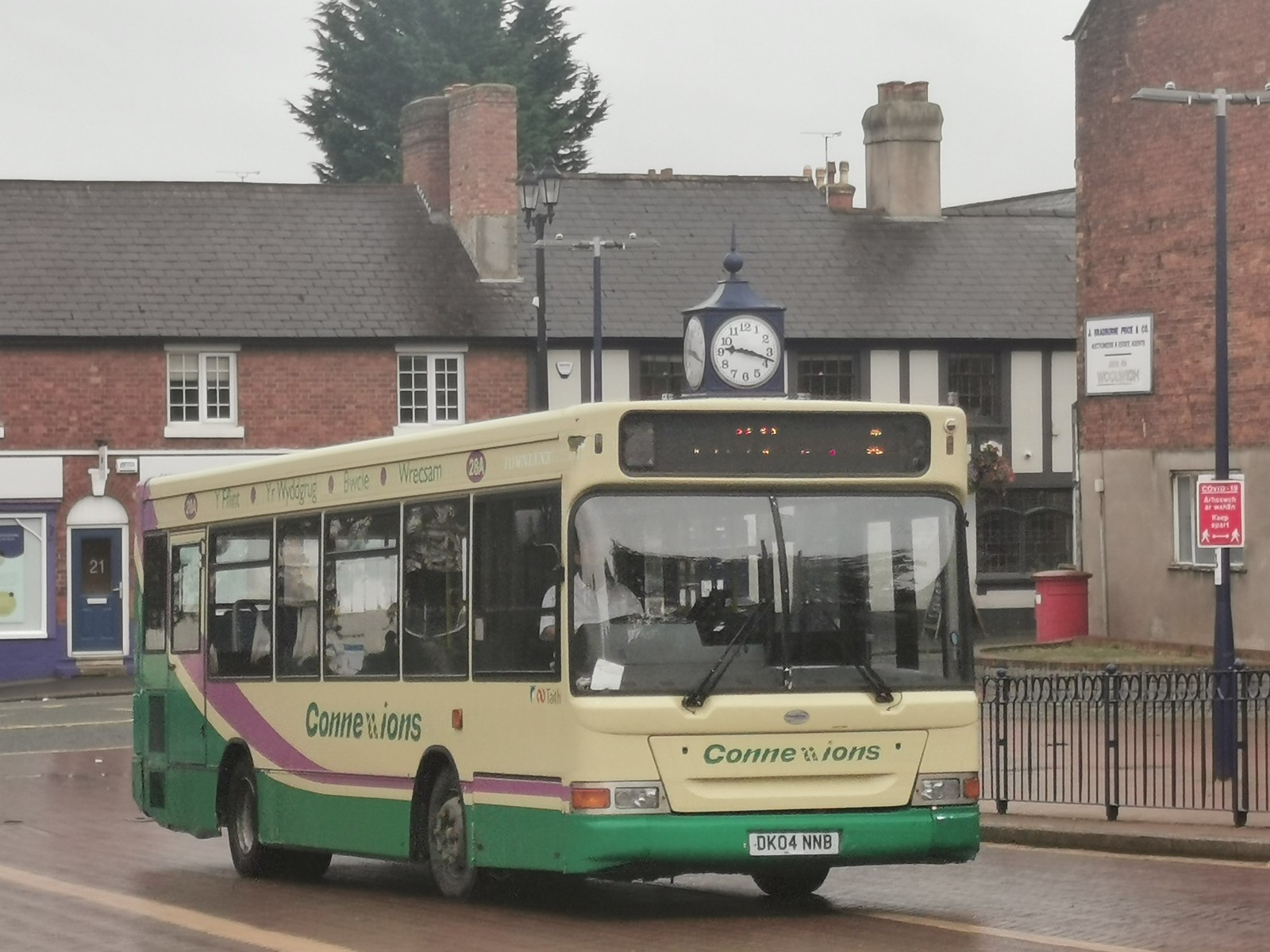The image depicts a light yellow transit bus on a gloomy day, with a slight white tint enhancing the overall dreary ambiance. The bus features a horizontal black digital display above a large windshield, with some of its digits possibly burned out, displaying small yellow and pink lights that are difficult to discern. The windshield is bordered by a black frame and divided by a black bar, with both windshield wipers pointing towards the center. Just below the windshield is the word "CONNECTIONS" spelled out in green letters on the bus's grille, flanked by silver headlights with orange lights on their outer sides. The bus has a distinctive green trim along the bottom, which rises towards the rear half, and is complemented by a purple line running along its side. The number plate reads "DK-004-NNB".

To the right side of the bus, there is a curb next to a black metal fence and a red sign with white, indistinguishable lettering. Above the bus is an analog clock with a white face and black numerals, showing the time as 4:45 (hour hand at 9 and minute hand at 4). In the background stands a brick building with a brown shingled roof, featuring dual red brick chimneys in the center and a light gray concrete chimney on the right. Completing the scene, a large evergreen tree rises to the left of the chimneys, adding a touch of nature amidst the urban setting.